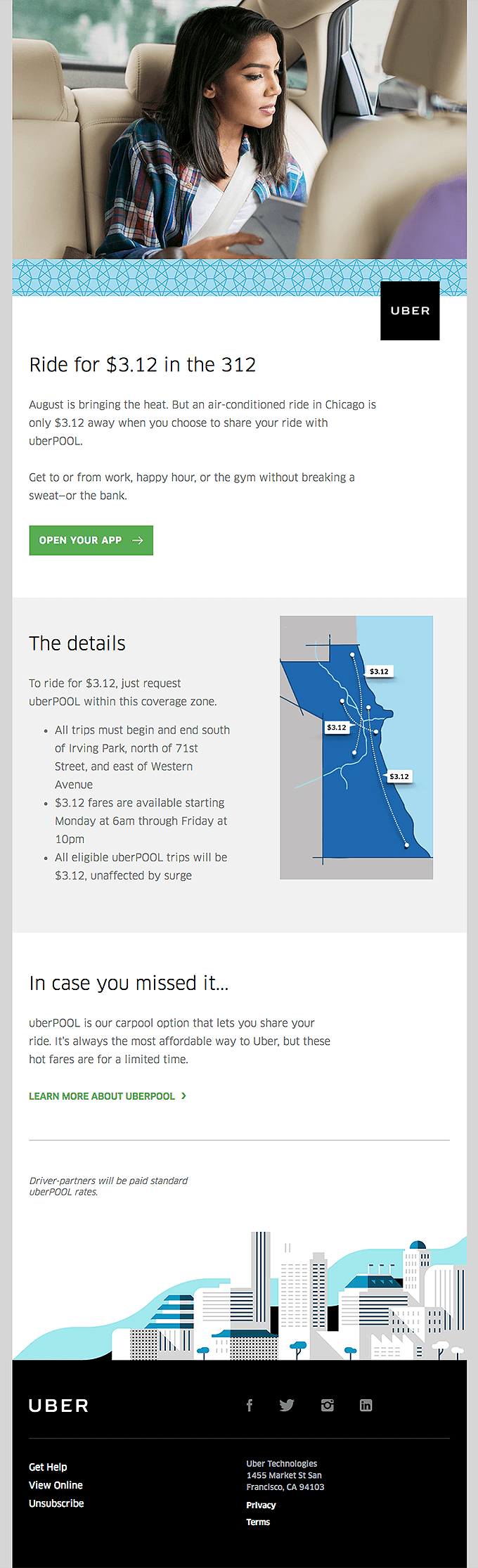**Image Description: UberPool Promotional Offer**

At the top of the screenshot is an image featuring a young woman with dark skin and shoulder-length dark hair, wearing a plaid button-up shirt. She is seated in the back of a tan interior car, secured with a seatbelt, and reading a book.

Below this picture, a blue bar spans across the screen, with the Uber logo on the right. To the left of the logo, in black text on a white background, it reads, "Ride for $3.12." The text continues, stating, "August is bringing the heat, but an air-conditioned ride in Chicago is only $3.12 away when you choose to share your ride with UberPool. Get to or from work, happy hour, or the gym without breaking a sweat—or the bank." An adjacent green rectangle indicates, "Open your app."

Following this is a gray bar with the heading, "The details." The instructions guide users to ride for $3.12 by requesting UberPool within a specified coverage zone. To the right of this text is a map shaded in blue, highlighting the coverage area. The bulleted points outline key details:
- All trips must begin and end south of Irving Park, north of 71st Street, and east of Western Avenue.
- $3.12 fares are available from Monday at 6 a.m. through Friday at 10 p.m.
- All eligible UberPool trips will be $3.12, unaffected by surge pricing.

Further down, against a white background, black text explains, "In case you missed it, UberPool is our carpool option that lets you share your ride. It's always the most affordable way to Uber, but these hot fares are for a limited time." In green text below, it says, "Learn more about UberPool."

A faint gray line separates this section from a line of black italic text stating, "Driver partners will be paid standard UberPool rates."

At the bottom of the image is a drawing of a city skyline with a blue wave behind it. The lower portion of the screenshot is a black band with text reading, "Uber," followed by options for "Get help," and instructions for online help and unsubscribing. Information about Uber technology and its address, 1455 Market Street, San Francisco, California 94103, is also provided, along with links to "Privacy" and "Terms."